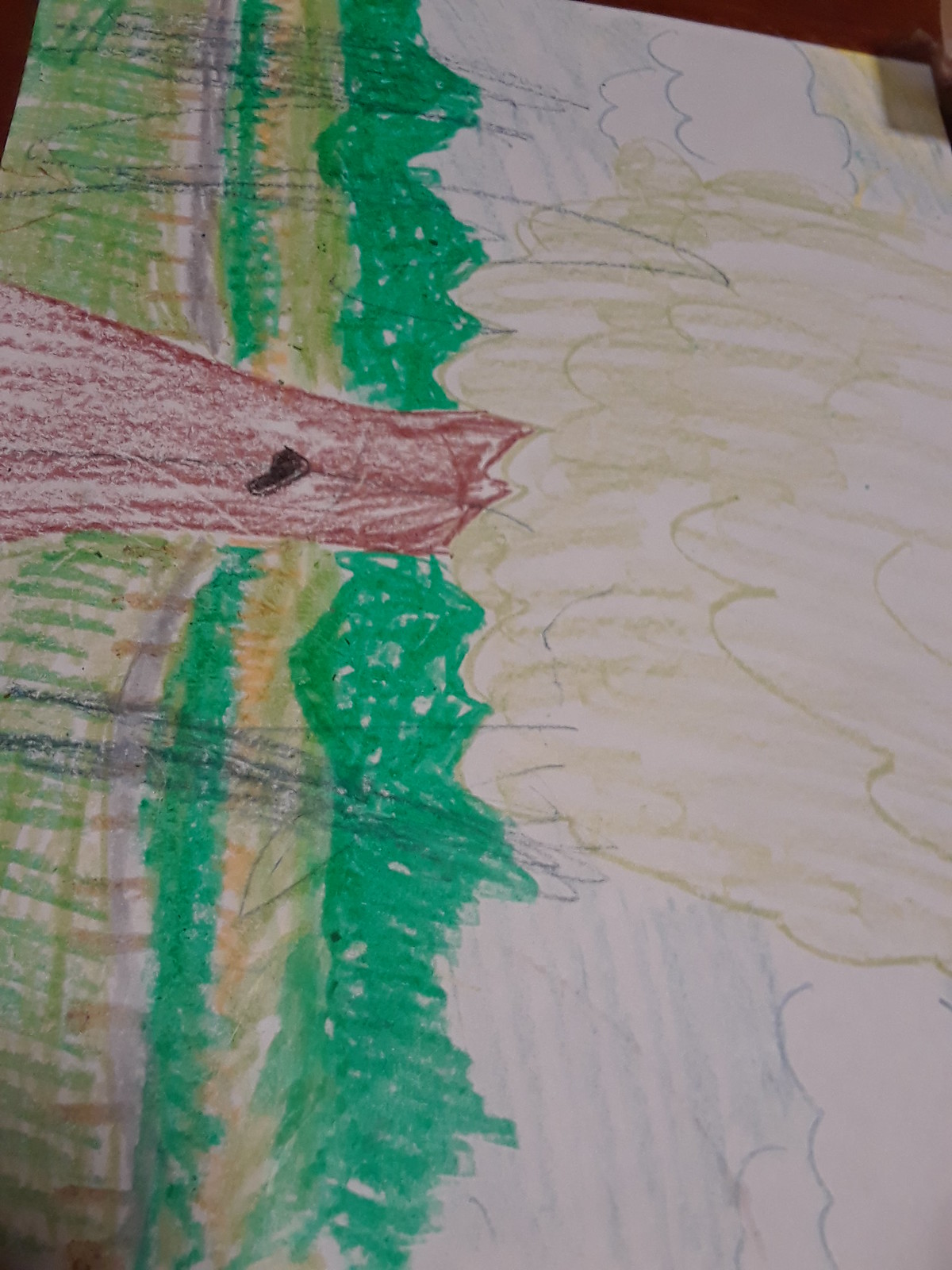This image resembles a child's painting, currently positioned sideways. To fully appreciate it, one must tilt their head. Dominating the foreground is a reddish-brown tree stump, textured with upward strokes. Nearby, stick-like figures, potentially representing plants, rise sporadically. At the center, a grey form could either be another tree stump or a fence post. Surrounding these elements is a vibrant green area, transitioning into a more subdued yellow-green, likely forming a hedge. The entire composition is characterized by vertical and horizontal lines. Above the hedge, a vivid green hue melds with a yellow-green, possibly indicating treetops, lending a sunny feel to the scene.